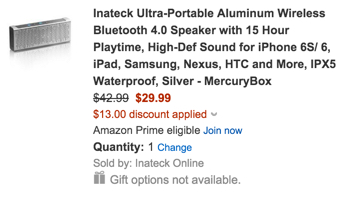This cropped screenshot from Amazon showcases an item for sale: a sleek, silver, rectangular object, identified as the Inateck Ultra-Portable Aluminum Wireless Bluetooth 4.0 Speaker. Positioned to the left of the item description is a photograph of the speaker, highlighting its compact and polished design. 

The detailed text beside the image describes the speaker's standout features, including its 15-hour playtime and high-definition sound quality, which are compatible with various devices such as iPhone 6s, iPad, Samsung, Nexus, HTC, and more. Additionally, the speaker is noted for being IPX5 waterproof. 

Initially priced at $42.99, the cost has been reduced to $29.99, reflecting a $13 discount. The product is Amazon Prime eligible, with an invitation to join the service. The default quantity is set to one, with an option to change it. The item is sold by Inateck Online, and gift options are not available, indicated by a small gray gift box icon with a ribbon bow. 

The image features a white background and contains no people, animals, plants, flowers, or trees.